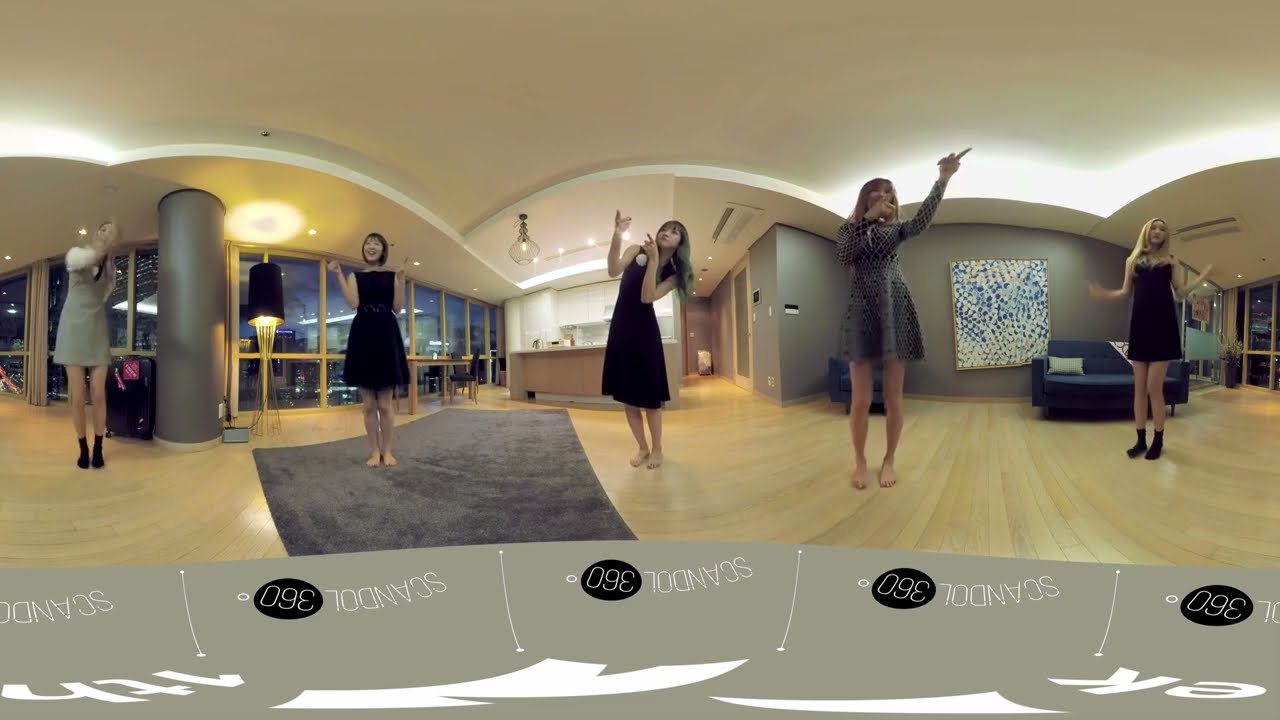The image depicts a large, modern room with a hardwood floor and a central gray carpet. The room's walls are painted gray and feature large windows. There is a noticeable painting with blue and white dots and a blue couch visible in one corner. The photo appears to have been captured and manipulated using a 360-degree tool, indicated by a watermark reading "Scandal 360" at the bottom of the image. The photo stitching creates a seamless panoramic view. Within the space, five women are performing a dance or sketch, their images repeated across the frame. They are dressed in various dresses, with most in black while a few wear patterns. The light fixtures hanging from the ceiling add to the modern aesthetic of the room. The image measures about 8 inches wide by 5 inches tall and is of medium quality.